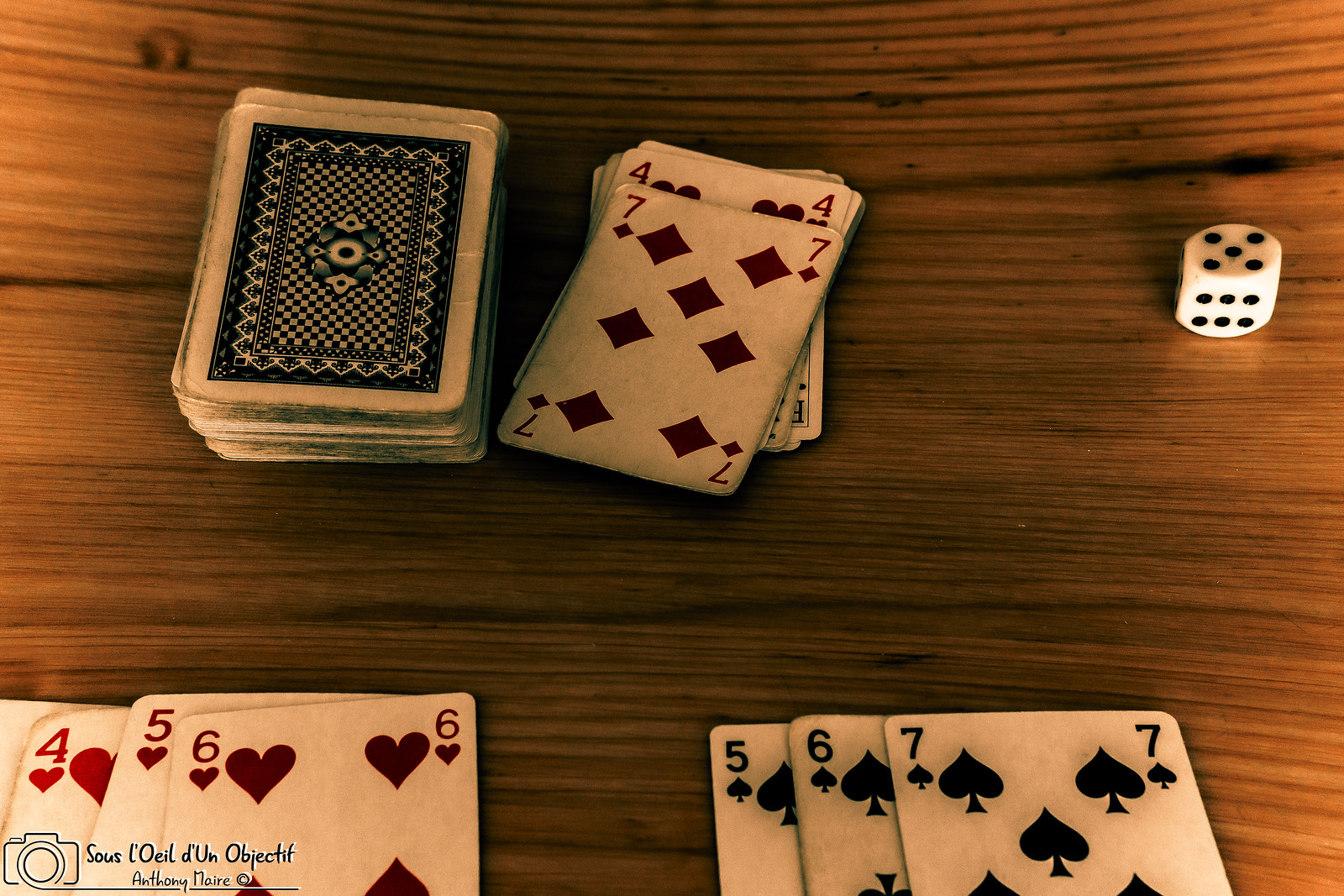A deck of well-worn playing cards is scattered on a wooden table. Some cards lie face down in a pile, while others are face up in smaller groups. One pile shows the 4, 5, and 6 of hearts, and another has the 5, 6, and 7 of spades. A single die, showing the number 5, rests nearby. The face-up cards in the larger pile include the 7 of diamonds and 4 of hearts, indicating that the players are using a full deck, although the exact game remains unclear. The photograph, taken by Anthony Amore and marked with a copyright notice in French at the bottom left ("Sui ou lai d'un objectif"), captures a mix of light and shadow cast over the cards, along with the shadow of the photographer. The edges of the cards are bent, suggesting frequent use.